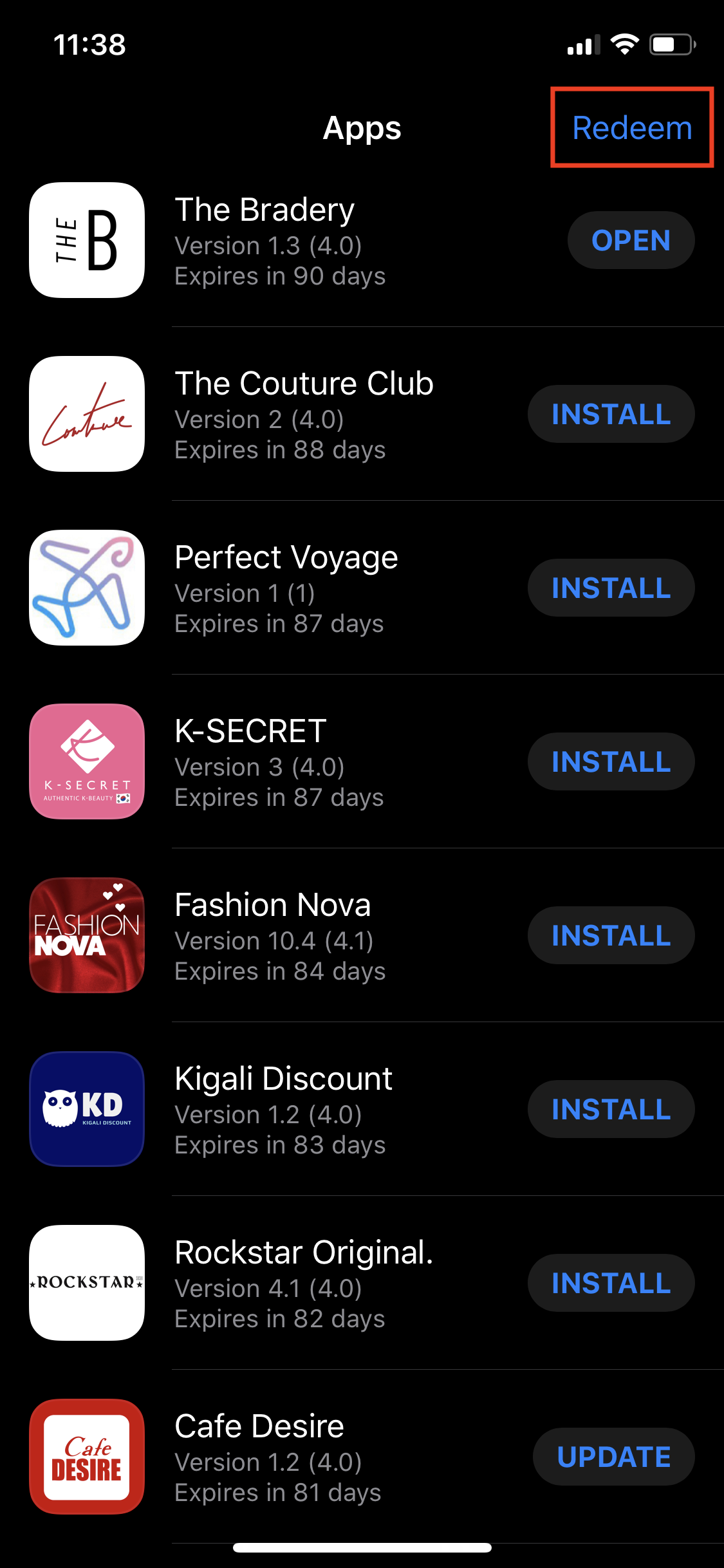A detailed depiction of the screenshot reveals a phone screen set against a black backdrop, illustrating a segment of an app store interface. At the very top, the screen displays the time as 11:38 in white text on the left, with indicators for service, Wi-Fi, and battery life on the right. Just below this top bar and centered is the word "Apps" in white, accompanied on its far right by the word "Redeem" in blue, enclosed within a sharpened red box.

Following this, a list of apps appears in organized rows. On the right side of each row, respective actions indicate their current status: the first app is marked "Open" in blue, while the remaining ones are labeled "Install." Notably, the bottom app instead shows "Update," all consistently in blue. The apps listed from top to bottom include: The Braidery, The Couture Club, Perfect Voyage, K-Secret, Fashion Nova, Kigali Discount, Rockstar Original, and Cafe Desire. Each app entry is coupled with version numbers ranging from 1 to 10.4, along with respective expiration periods in days.

The left side of the screen showcases the app icons, rendered in various thematic designs:
- The Braidery's icon features a capital "B" in black text on a white background.
- The Couture Club displays "Couture" in red on a white background.
- Perfect Voyage symbolized by an airplane icon against a white background. 
- K-Secret includes the text "K-Secret, Authentic Beauty," alongside an image of the South Korean flag with a pink "K" contrasted on a white and pink backdrop.
- Fashion Nova presents its name arrayed in white text on a vibrant red background.
- The KD app sits within a blue background.
- Rockstar Original is placed on a white canvas.
- Cafe Desire is showcased in red text against a white background, bordered in red.

This comprehensive layout incorporates intricate visual and textual details, encapsulating the essential information presented in the screenshot.